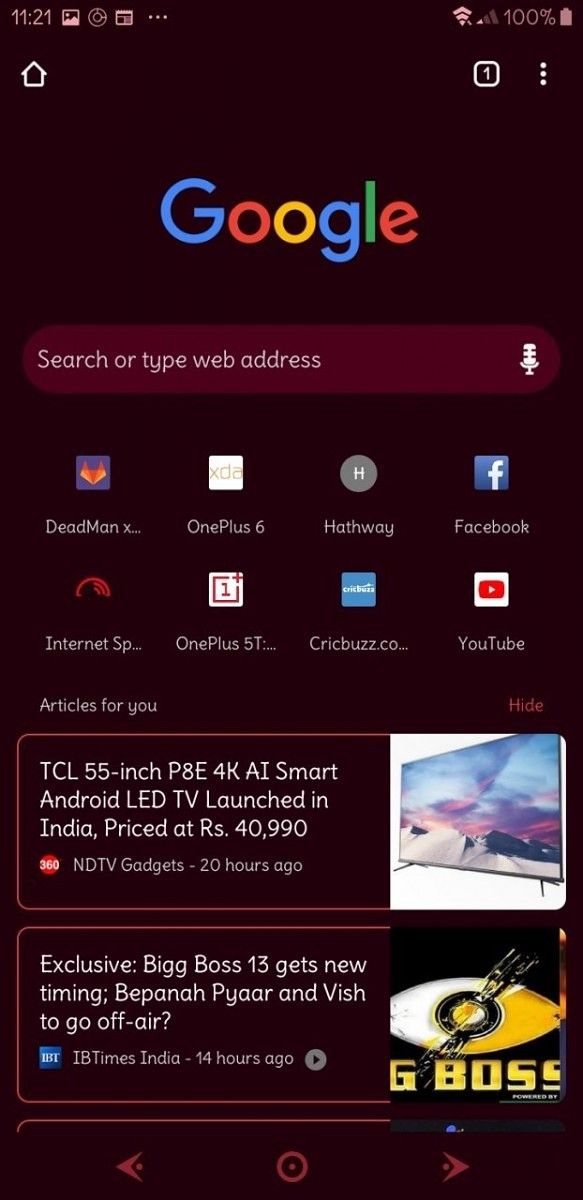This is a detailed screenshot from an Android device captured at 11:21 AM. The device shows a full battery at 100% and is connected to Wi-Fi. The user has saved several websites as bookmarks, including YouTube, Facebook, Hathaway, QuickBuzz.com, and four others, making a total of eight bookmarked sites that are visible. Below the bookmarks, two articles are displayed. The first article is about a newly launched AI smart TV priced at 40,990 rupees, sourced from NDTV, suggesting the user is likely based in India, as NDTV is a local news outlet. The second article discusses changes to the timing of Big Boss Season 13, published by IB Times India. This detailed view offers insights into the user's interests and browsing activity.